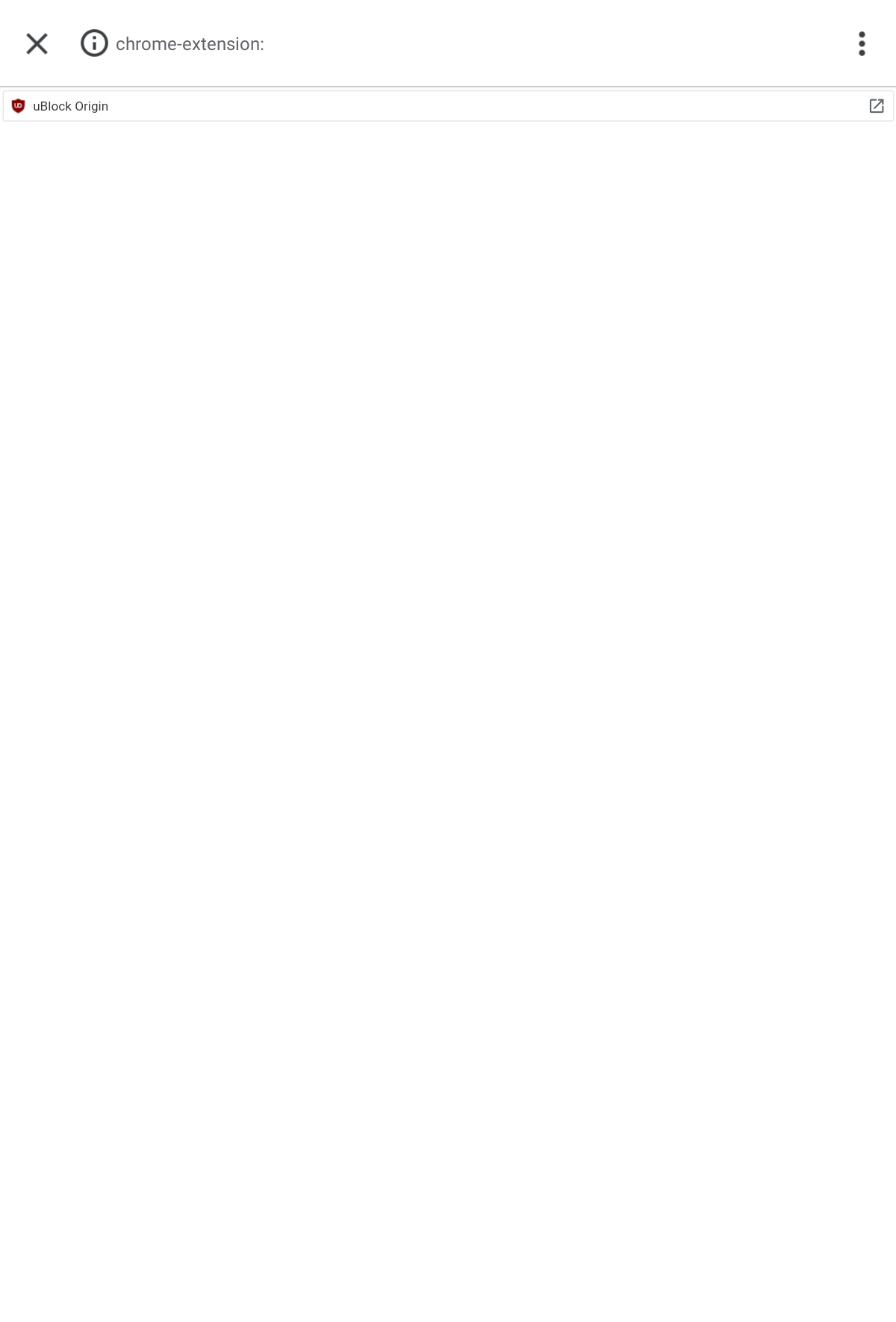This image is a narrow, left-to-right horizontal strip with a white background, blending seamlessly into the white display of the computer screen. The minimalistic interface suggests that it is part of a web browser extension, specifically within a settings or options menu on a less informative webpage.

Detailed Description:

- **Top Left Corner:** A muted, dark gray 'X' icon, presumably for closing or dismissing a window or dialog box.
- **Next to the 'X' Icon:** A circled 'i' icon, representing an information button.
- **Following the Icons:** The text "Chrome-extension:" indicates that the visual content pertains to a Chrome browser extension. 
- **Far Right (Aligns Vertically):** Three vertical dots, a common symbol for additional options or a menu, positioned after a long horizontal line that separates sections.
- **Separator Below:** Underneath the previously mentioned horizontal line, there is a small icon alongside the text "uBlock Origin," identifying it as part of the uBlock Origin extension interface.
- **Adjacent to uBlock Origin:** There appears to be an interactable element (such as a button or link) on the far right, aligned with the prior elements, also separated by another long horizontal line below.

The elements and layout suggest a simplified and minimal design, focused on essential icons and text without additional graphical contexts.